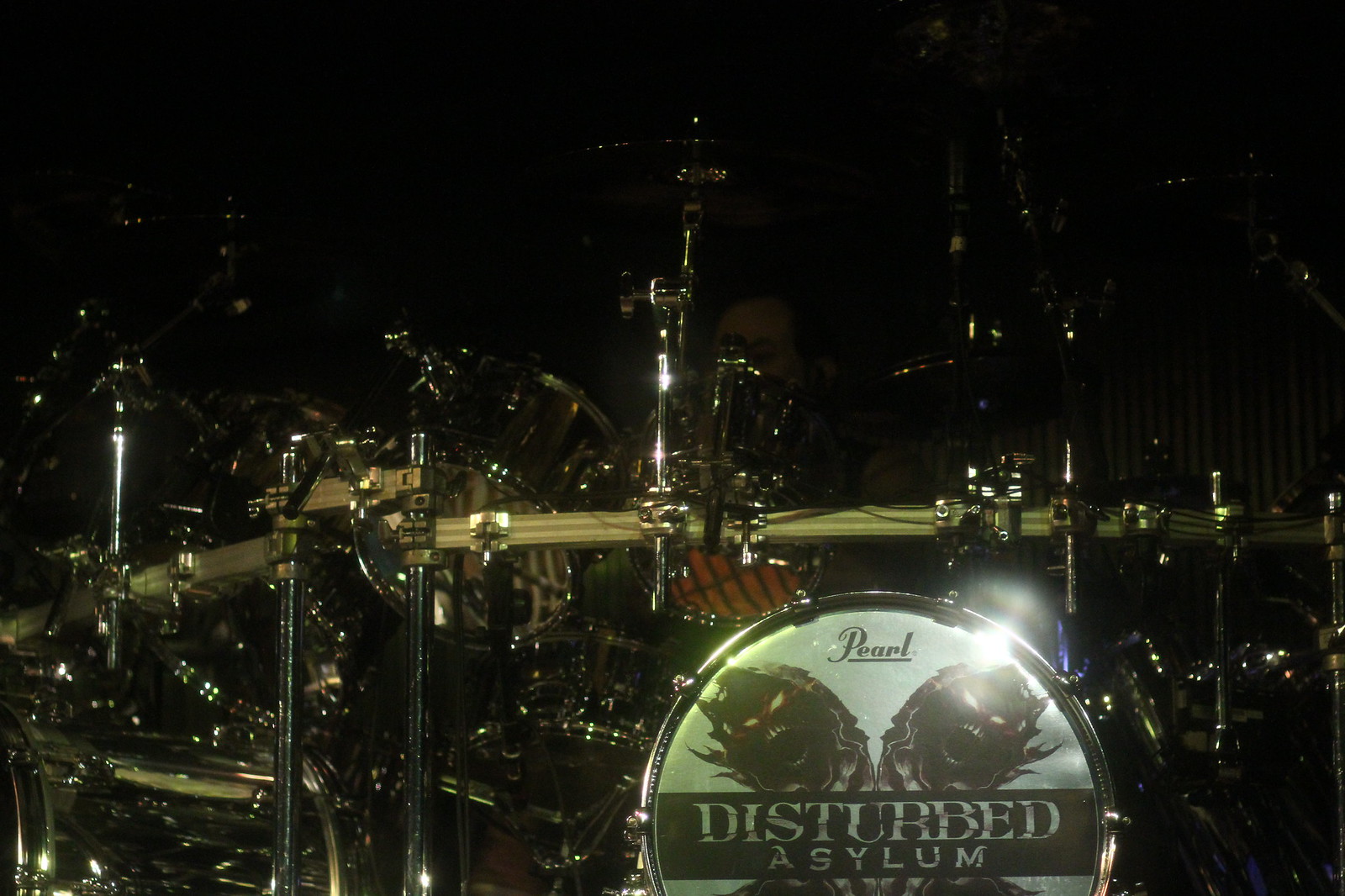In the dark, enigmatic photograph, a large, chrome-heavy drum set shimmers under a faint light, drawing the eye to its reflective surfaces. The centerpiece is a bass drum prominently featuring the logo "Pearl" at the top, with vivid, stylized white text beneath reading "Disturbed Asylum." This text is set against a black background and flanked by eerie, death-like faces with glowing eyes. The intricate network of interconnected drums and metallic fixtures gleams, casting sparkles across the image. Behind the drums, a shadowy figure—a drummer—sits partially obscured, with only part of their face visible, illuminated just enough to reveal a solitary eye. The photo's upper portion remains engulfed in darkness, adding an element of mystery around the faintly discernible drumming figure.